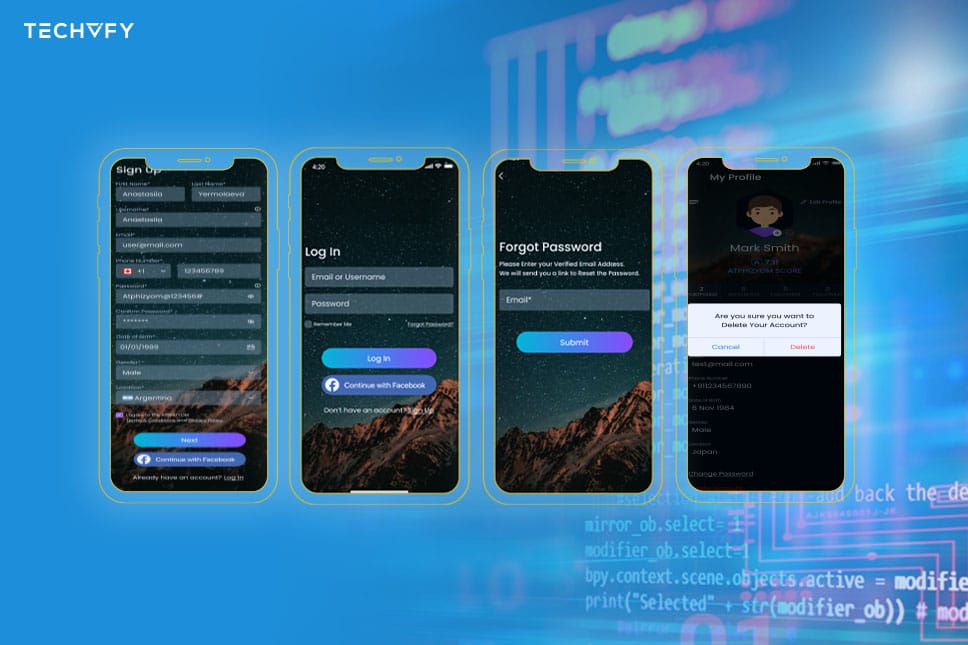This composite image, titled "Techify," features a main image in the upper left-hand corner with the "Techify" logo prominently displayed. Arranged in a left-to-right sequence, there are four smaller images, each depicting different screens of a mobile phone. The first phone screen displays a "Sign Up" interface, and the second phone showcases a "Log In" screen. The third phone presents a "Forgot Password" prompt. Each of these three screens is set against a serene nighttime mountain backdrop, with twinkling stars visible in the sky. In contrast, the fourth image diverges from the mountain theme, instead featuring a user profile screen overlaid with a critical notification that asks, "Are you sure you want to delete your account?" It provides options to "Cancel" or "Delete." The primary background of the main image is a calming blue, and an intriguing snippet of code resides in the lower right-hand corner, hinting at the tech behind the scenes.